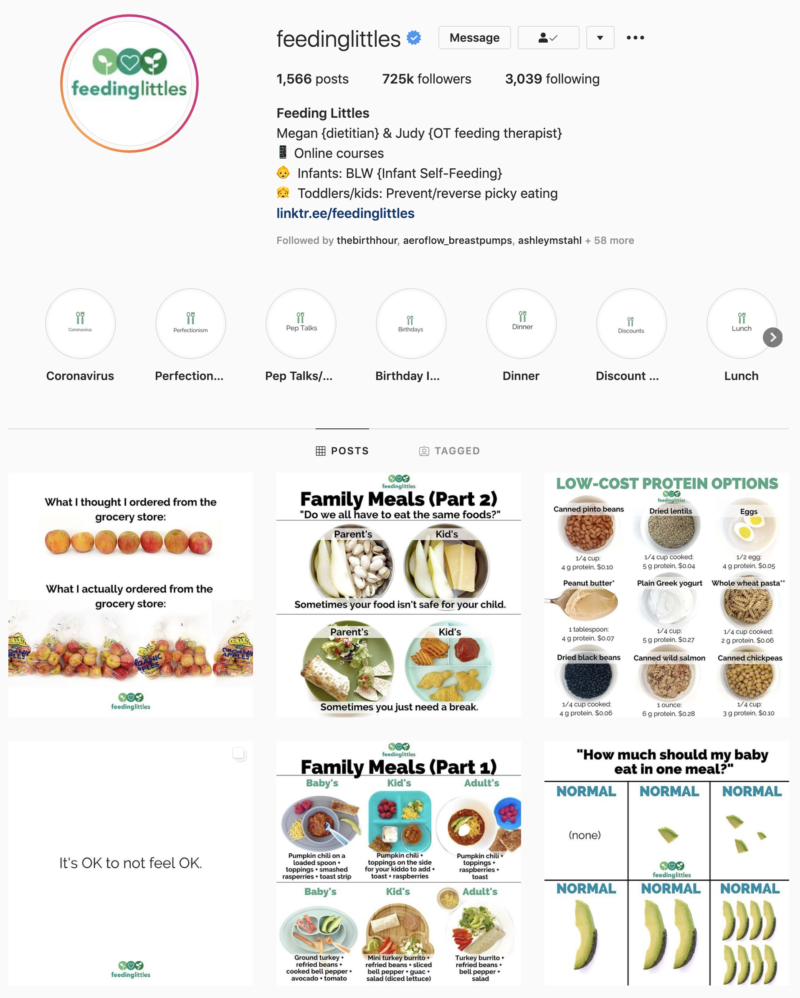Here's a cleaned-up and detailed caption for the described image:

---

This Instagram screenshot features the account of 'Feeding Littles'. The profile has posted 1,566 times and boasts a significant following of 725,000 followers, with the account following 3,039 others. A small icon indicates that you are currently following this account. In the top-right corner of the profile, there are three dots for additional options.

The account is managed by Megan, a Dietitian, and Judy, an Occupational Therapist (OT) specializing in feeding therapy. Feeding Littles offers online courses focused on infant and toddler nutrition. Their bio includes a clickable link to further resources and mentions being followed by prominent figures.

Highlighted story sections include 'Coronavirus Perfection', 'Pep Talks', 'Birthday Dinner', and 'Discount Lunch'. 

The main feed displays six visible posts, which cover various topics such as 'Family Meals, Part Two', 'Low-Cost Protein Options', 'Bananas: What's Normal?', 'How Much Should a Baby Eat?', and more. These posts provide valuable information on toddler meals and the emotional reassurance that "It's okay to not feel okay."

---

Note: Some of the contextual arrangements and specific word choices have been provided to ensure the caption is informative and structured, based on the verbal description.